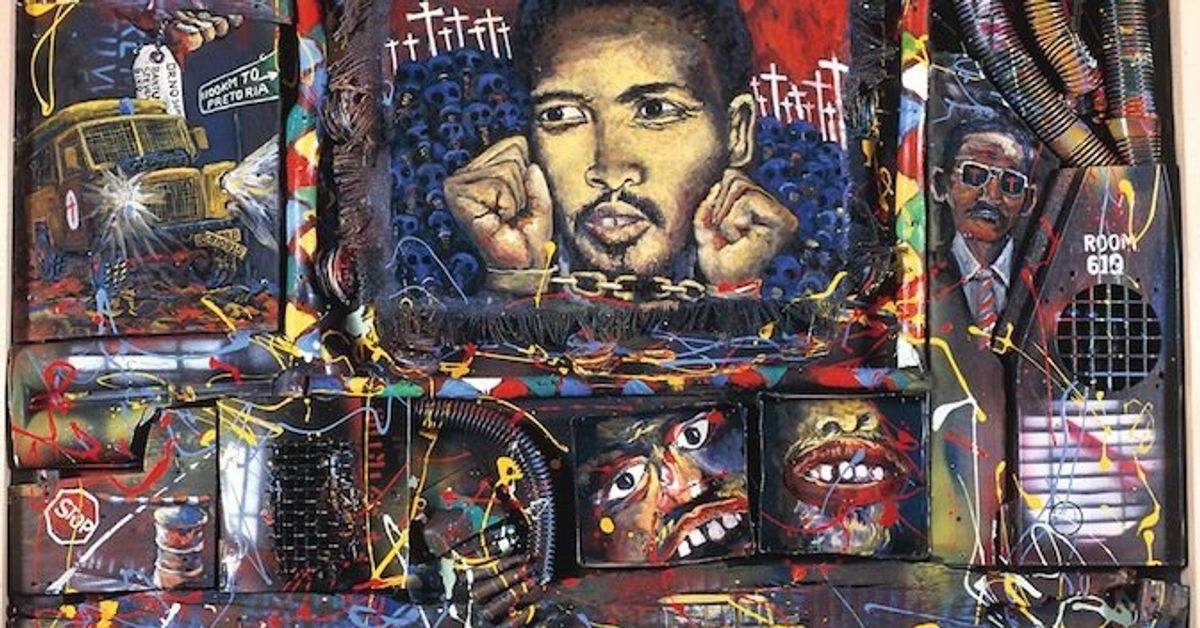The photograph captures an intricate, large-scale mural painted on the side of a building. The mural's complex artistry combines various styles and themes, making it a vivid tapestry of visual elements. 

On the top left corner, a school bus is depicted, armored in an apocalyptic style, adding a dystopian touch. Below this bus is a broken stop sign, further contributing to the chaotic atmosphere. The mural's central and most striking feature is an African-American man in handcuffs, surrounded by dark, ghostly figures or zombies, creating a haunting and evocative scene. The backdrop behind these figures is filled with rows of white crosses, set against a deep, dark crimson sky, which intensifies the ominous mood.

On the bottom portion of the mural, random splotches of paint in blue, red, white, and green add to the mural's vivid and chaotic aesthetic. Additionally, there's a stop sign and a barrel painted near the bottom left.

Further right, another African-American man is depicted, wearing sunglasses that reflect the white crosses behind him, offering a sense of depth and layers within the artwork. The mention of "room 619" indicates a probable connection to a specific location or event, possibly signifying elements of protest or social commentary.

Overall, the mural appears to be a powerful statement on African-American struggles and resilience, blending symbolic elements of chaos, protest, and hope through its diverse and vivid artistic expression.